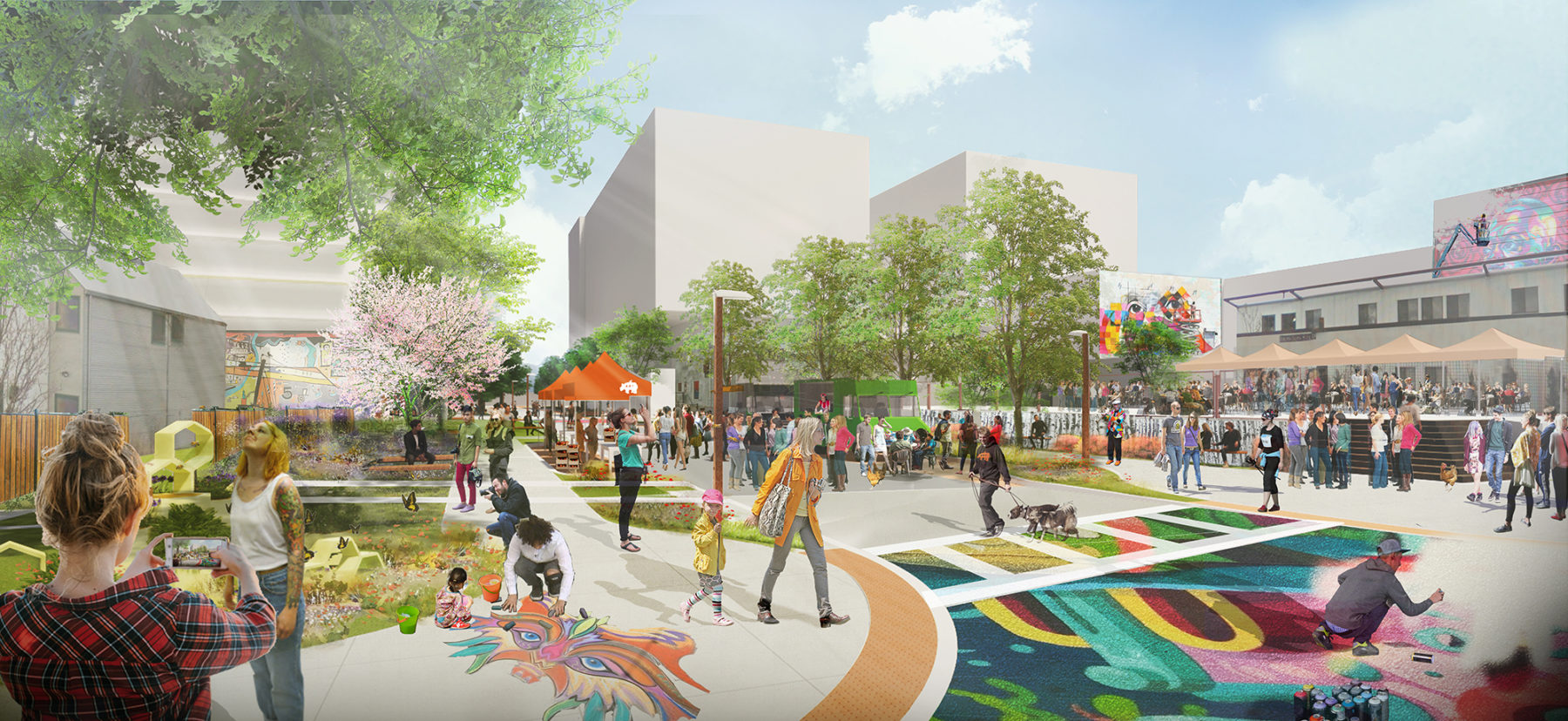The image showcases a vibrant computer rendering of a bustling urban public space brimming with activity. In the left part of the frame, a woman captures a photograph of another woman who is gazing up at a cherry blossom tree, creating a whimsical atmosphere reinforced by the flowering tree's delicate branches. Children enthusiastically draw a Mardi Gras mask-like illustration on the pavement beneath them. Nearby, a cluster of orange pop-up tents draws attention with a large group of people gathered around them, while others meander in the background.

Toward the right, a man sporting a red hat walks his two black-and-gray dogs across a brightly colored rainbow crosswalk. An artist, situated further to the right, is engrossed in painting what appears to be a public mural. This mural features a large, vibrant wolf in hues of orange, light purple, and turquoise, capturing the imagination of onlookers. The demographic diversity is evident with a mix of families and individuals from various backgrounds, creating a microcosm of community life. The scene is bustling and diverse, celebrating art, nature, and human connection.